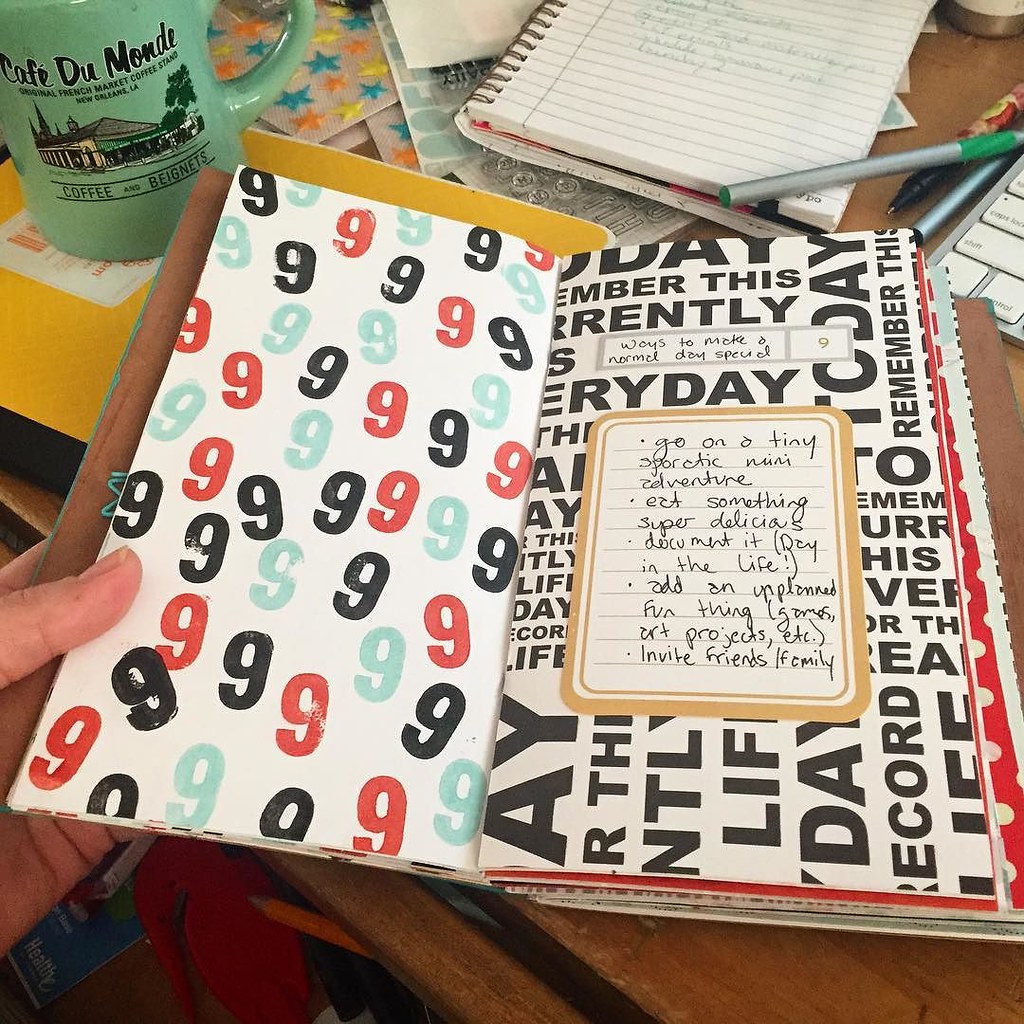In this photograph, a person is holding open an illustrated journal with their left hand. The journal is filled with decorative elements, and the current page is titled, "Ways to Make a Normal Day Special." The page features a blank square decorated with large sans serif text that reads: "go on a tiny sporadic mini adventure, eat something super delicious, document it, a day in the life, add an unplanned fun thing like games, art projects, etc., or also invite friends and family." The opposite page appears to be adorned with a bunch of colorful numbers, primarily nines, randomly stamped in black, red, and blue without any discernible pattern. 

The journal rests on a cluttered writer's desk. In the upper left corner, there's a white coffee mug with "Cafe du Monde" written in black font. Nearby, in the upper right corner, an open spiral notebook with a pen lies on top, partially covering a sliver of a laptop. The desk is scattered with various items, including papers, possibly stickers, and additional writing tools, embodying the creative chaos of an active workspace.